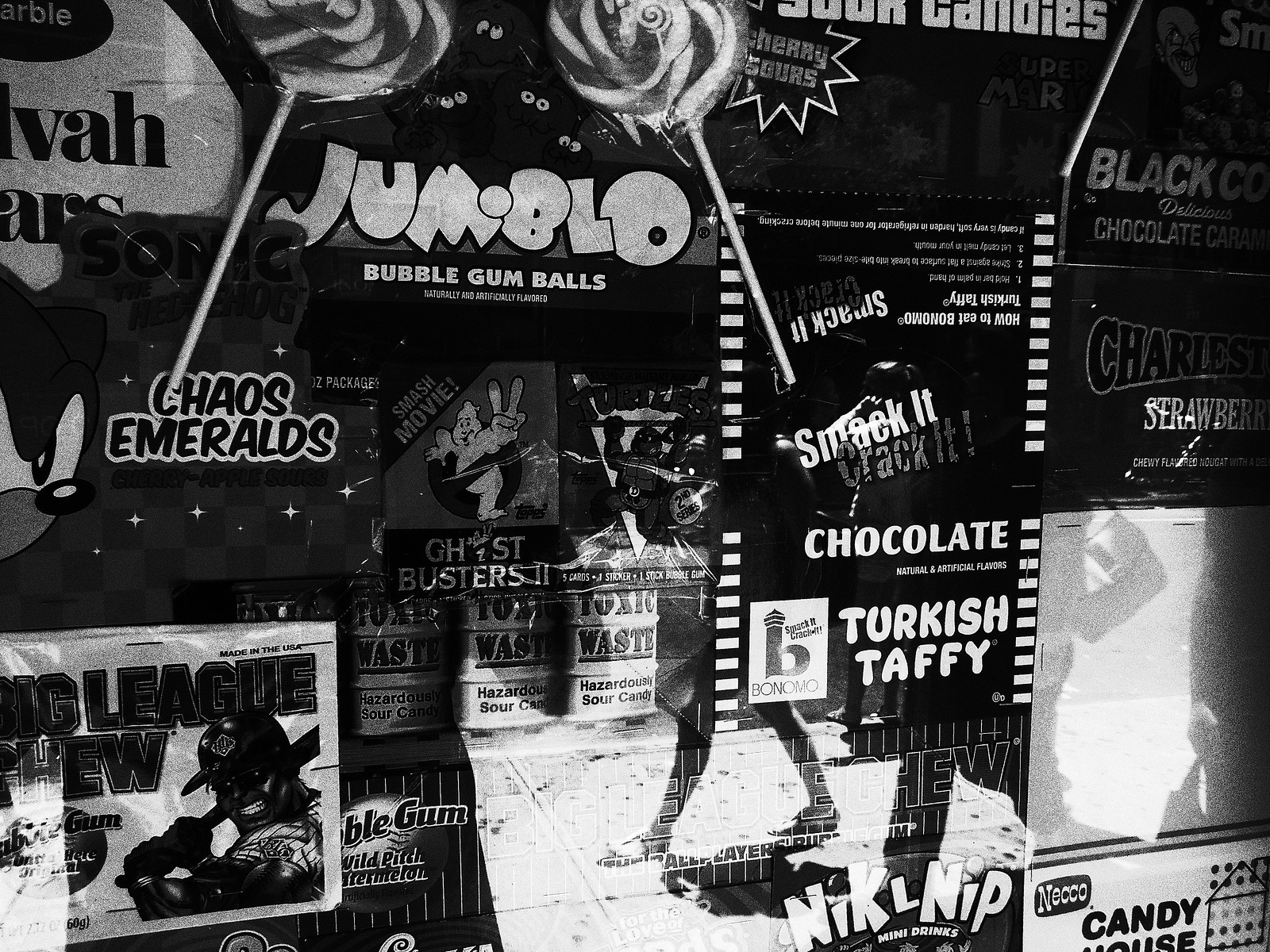This black-and-white image appears to depict the storefront of a nostalgic candy shop, possibly from around 1990. The stark contrast between the blacks and whites gives the scene a timeless quality, emphasizing the various reflections of people walking on the sidewalk and casting shadows in front of the store. The storefront window is filled with an array of candy advertisements and logos, creating a vibrant yet monochromatic display. 

Prominent in the window are items like Big League Chew bubble gum, easily identifiable by the black-and-white packaging featuring a baseball player. Nearby, signs advertise Jumblo bubblegum balls and Chaos Emeralds, all in cartoonish lettering that evokes a playful atmosphere. Additionally, the window features references to popular culture from the era, such as a Sonic the Hedgehog sign and T.O.P.S. cards for "Ghostbusters 2" and "Teenage Mutant Ninja Turtles."

Recognizable candy brands include Turkish Taffy, Charleston Chew, Nick-a-Nip, and Smack It, Crack It chocolate. The shop is named "Candy House," catering especially to children, with various items like large lollipops and sour candies, adding to the allure. The reflective surface of the glass enhances the nostalgic feel, capturing the essence of a simpler time when such stores were a delight for kids. The detailed assortment of candies, gum, and cultural memorabilia makes this image a charming snapshot of a bygone era.